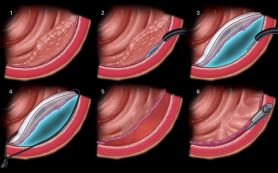A highly detailed, close-up medical infographic set against a black background comprises six sequential images labeled 1 through 6, arranged in two rows. These visuals depict the progressive steps of a surgical procedure, likely the removal of a growth or foreign body from a section of tissue. Each image is shaped like a tapered section, with a red curved line at the base and a pink interior showcasing multiple curved lines and what appears to be muscle or other body tissue. 

1. The first image shows the initial state of the tissue.
2. The second image introduces a small black hose injecting a neon blue substance above the red line.
3. The third image reveals the tissue filled with this blue substance, possibly indicating a diagnostic contrast or marking fluid.
4. The fourth image highlights the removal of the tool, leaving the blue substance intact.
5. The fifth image depicts the blue substance changing to a maroon color, perhaps indicating a reaction or solidification phase.
6. The sixth image shows another tool inserting, seemingly to remove the now hardened blue substance, illustrating the final step of the procedure with the affected area cleared and the tissue starting its healing process.

Throughout the sequence, a neon blue substance plays a pivotal role, transitioning colors and states to reveal the methodical approach to addressing the tissue anomaly. Each step is meticulously illustrated, showing the intricate process from diagnosis to the surgical removal of the growth, capturing the essence of the medical procedure in stunning detail.